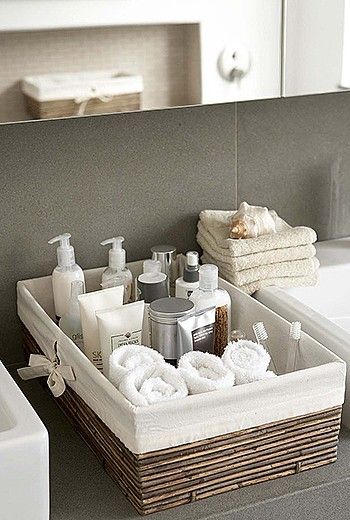In this upscale bathroom setting, possibly found in a high-end private home or luxury hotel, a close-up image captures a meticulously arranged wicker basket filled with various toiletries. The basket, a rich dark brown with a linen insert draping over its sides, is positioned elegantly between two pristine white sinks. Within it, an array of items is neatly stored, including several push-bottle creams, tins, and jars holding transparent toothbrushes that stand upright. Additionally, four face cloths, rolled neatly into spirals, enhance the organized appearance.

A large mirror, mounted on the wall, reflects the opposite side of the bathroom, revealing a similar basket and further extending the sense of symmetry and order. The dark grey tiles beneath and behind the basket add a touch of sophistication to the space. To the right of the central basket, another stack of four face cloths, folded crisply into squares, serves as a base for an elegantly placed shell, contributing to the bathroom's luxurious ambiance.